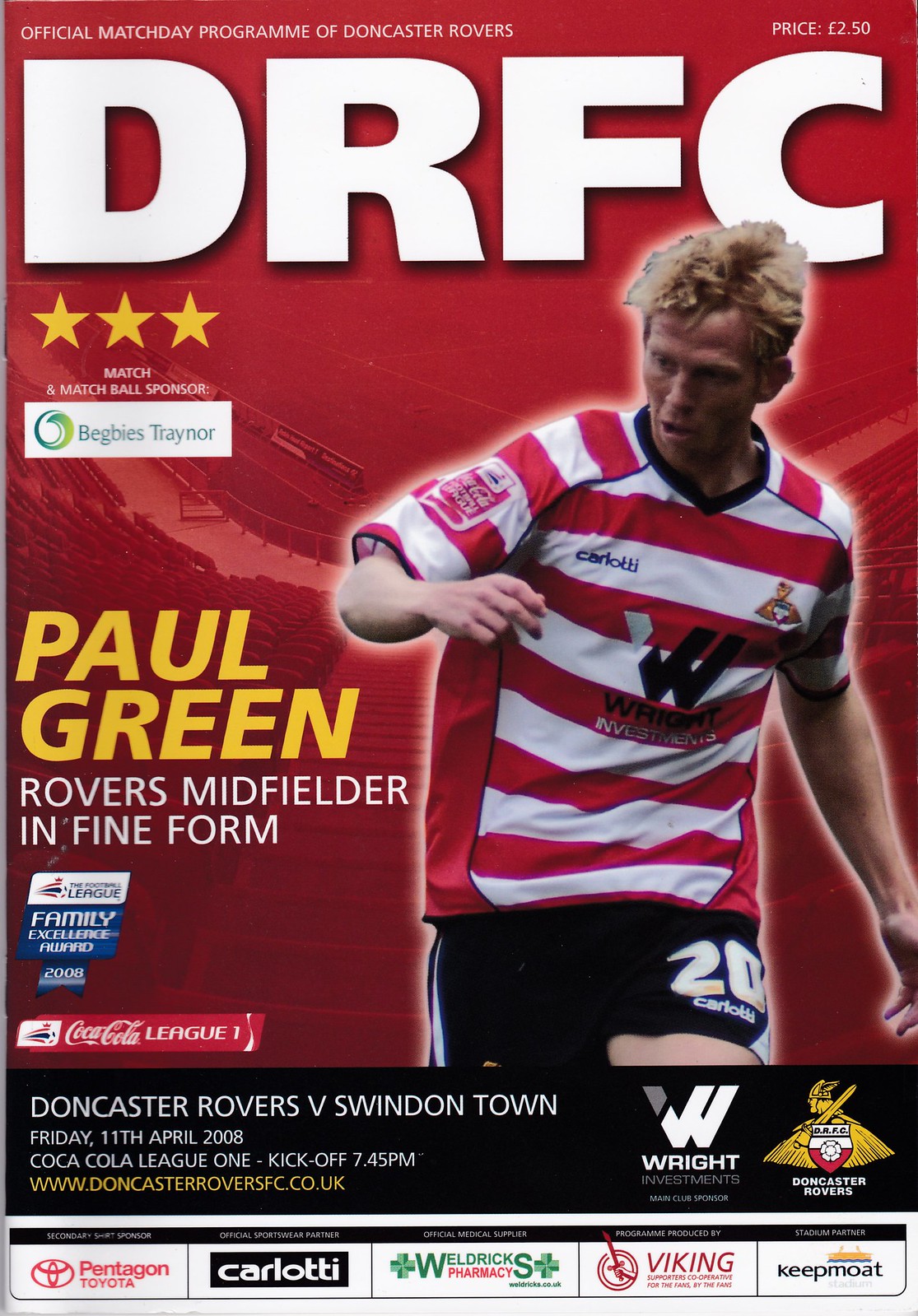This image is the front cover of a soccer magazine titled "DRFC." The background features a view of the stands of a soccer pitch, all colored in bright red. At the top, "DRFC" is prominently displayed in large white capital letters. The centerpiece is a silhouette of a Caucasian man with blonde hair, identified as Paul Green, wearing a red and white horizontally striped jersey with a black logo and black shorts with the number "20." To the left of the man, "PAUL GREEN" is written in large yellow capitalized letters, and just below it in smaller white text, it states, "Rovers Midfielder in Fine Form." A large black bar spans the bottom of the image with white text reading, "Doncaster Rovers v Swindon Town." Beneath that, in smaller text, it details, "Friday 11th April 2008, Coca-Cola League 1, Kick-off 7:45 p.m." Below this, the website "www.doncasterroversfc.co.uk" is written in yellow. Additionally, there are several sponsor logos at the bottom, suggesting affiliations with Pentagon, Toyota, Carlotti, Waltrix Pharmacy, Viking, and Keepmoat. The overall color scheme prominently features red, white, and black.